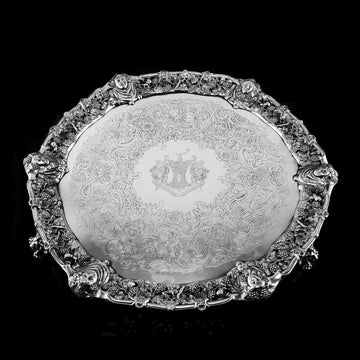The photograph showcases a highly ornate silver platter set against a stark black background, emphasizing its intricate craftsmanship. The platter features a raised, finely detailed border adorned with an elaborate array of carvings, including six distinct faces that add a sense of historical richness and grandeur. The surface of the tray is meticulously etched with geometric patterns and floral motifs, adding to the texture and allure. The centerpiece of the tray is a shiny, smoother oval area, which is less intricate but engraved, featuring a central emblem or family crest that is difficult to make out, suggesting a possible heritage or ceremonial significance. This silver platter, possibly part of a tea service or a display piece, combines artistic elegance with historical depth, making it a striking artifact.